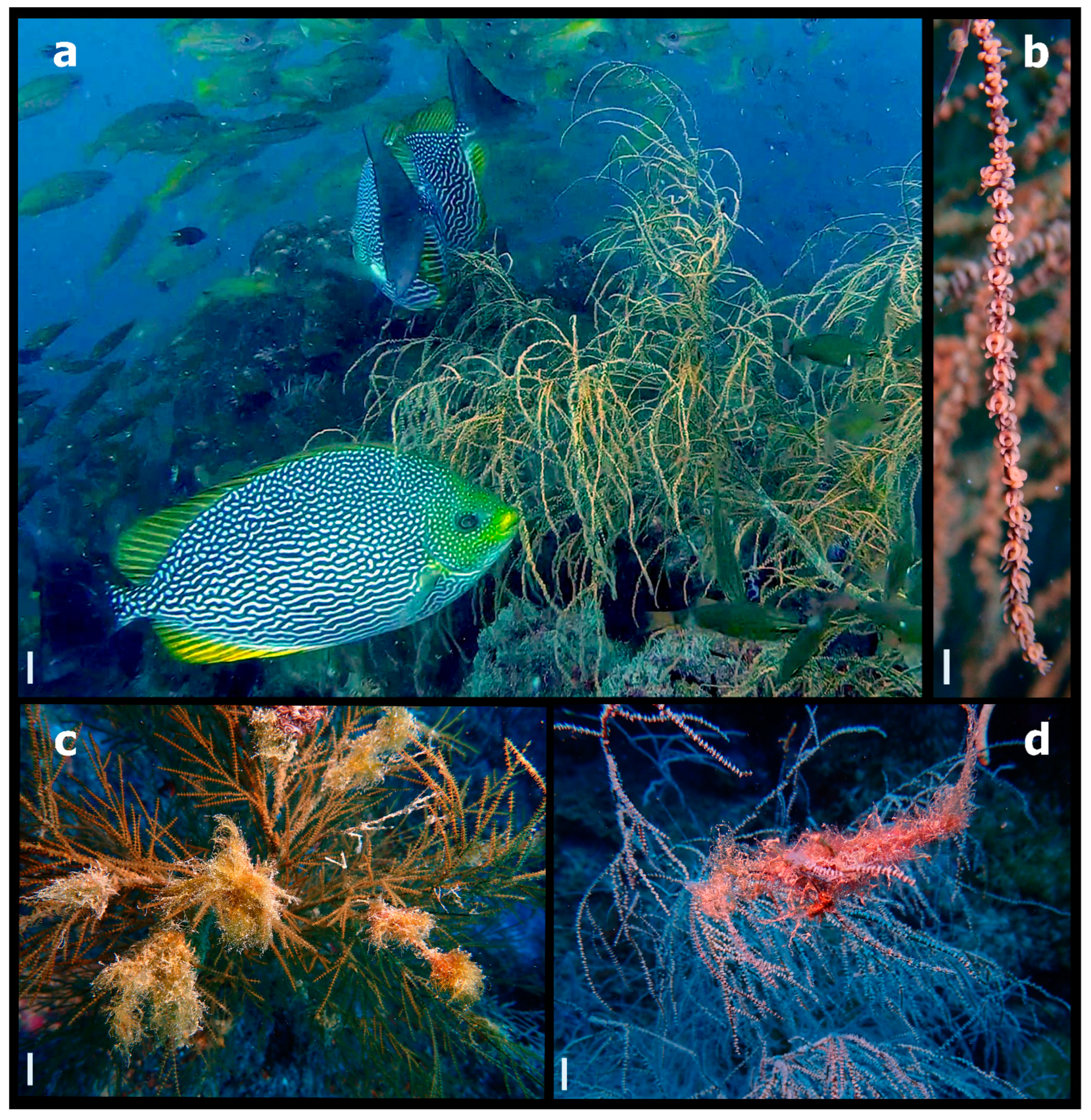The composite image consists of four distinct underwater photographs arranged in a 2x2 grid. The largest photograph, labeled "A" in the top left corner, dominates the top left quadrant of the grid. It captures an enchanting underwater scene featuring a striking blue, green, and white fish. The fish displays a pattern of white lines divided by thick black stripes across its body, with its face and fins tinged with a yellow-green hue. In the background, a school of similar fish swim in formation, and the scene is embellished with green sea grass and other aquatic plants. The blue water provides a serene backdrop.

The second photograph, labeled "B" in the top right corner, showcases a long vine of delicate pink plants, resembling coral. This strand of pink coral stretches vertically and is mirrored by similar corals in the background.

In the bottom left quadrant, labeled "C," there's an image of another underwater scene featuring a vibrant yellow brushy coral with thin, more golden extensions protruding from it. The blue water surrounds this distinct coral formation, enhancing its vivid colors.

Lastly, the bottom right photograph, marked "D," features a coral resembling the texture of the one in image "C," but this time in a striking red and blue coloration. The underwater background and the coral's vivid hues create a visually captivating conclusion to the series.